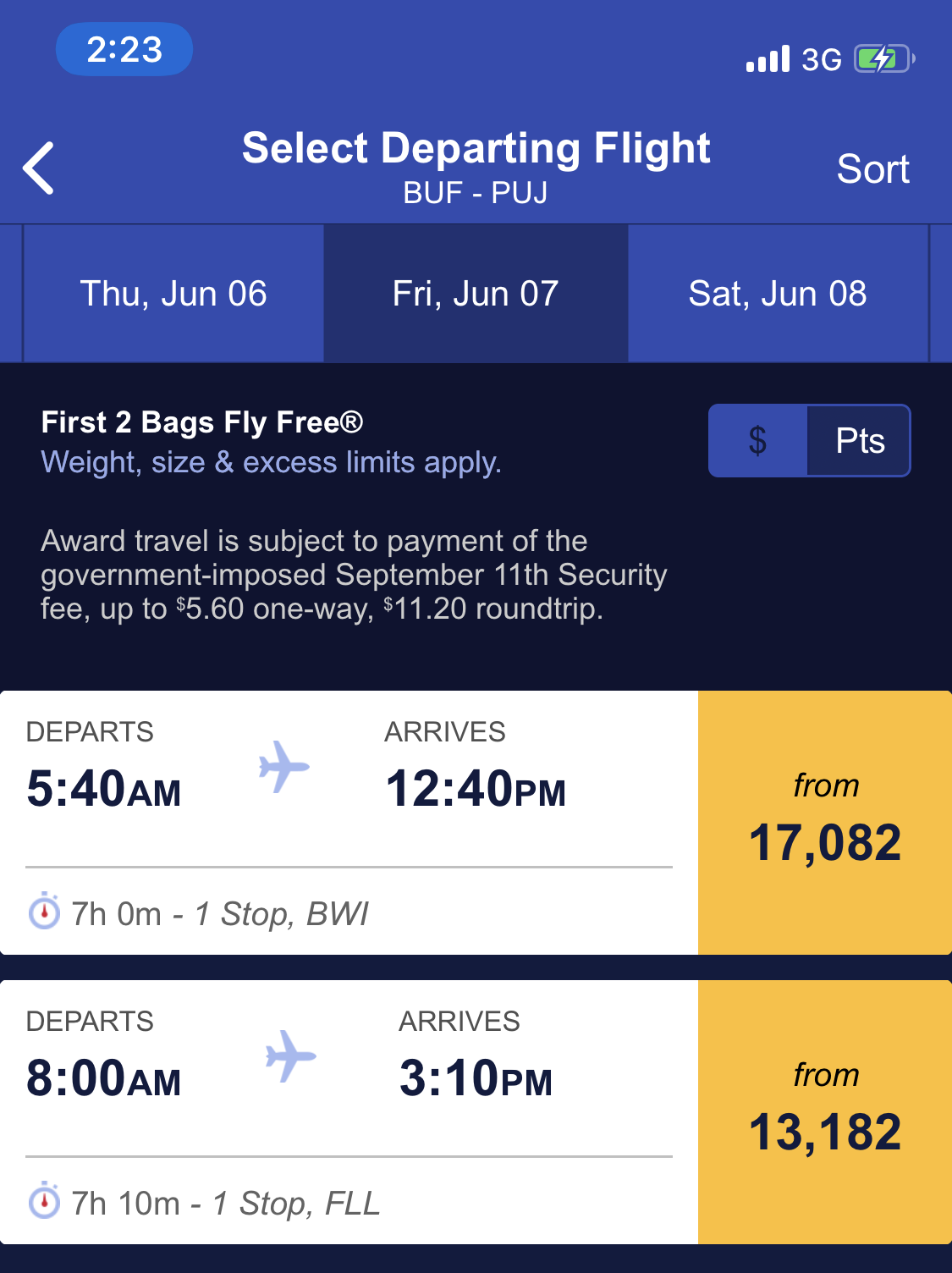The image showcases a mobile phone displaying a travel website. The phone is connected to a 3G network, showing a strong signal with three-quarters of its battery life remaining. The current time displayed is 2:23 PM.

The website on the phone has a blue banner at the top with the text "Select Departing Flight" in white font. The selected route is from Buffalo (BUF) to Punta Cana (PUJ). Users can sort the flights using a rightward arrow button labeled "Sort". 

Below the banner, dates are listed: Thursday, June 6; Friday, June 7; and Saturday, June 8; with Friday, June 7 highlighted. 

A notice states, "First two bags fly free; weight, size, and excess limits apply." There's mention of additional costs: "Award travel subject to payment of the government-imposed September 11 security fee up to $5.60 one-way, $11.20 round-trip."

Two flight options are provided:
1. Departure at 5:40 AM, arrival at 12:40 PM, priced from $178.20. 
   - Duration: 7 hours, 1 stop.

2. Departure at 8:00 AM, arrival at 3:10 PM, priced from $138.20. 
   - Duration: 7 hours 10 minutes, 1 stop.

Each flight detail includes a small dollar sign and point sign indicating pricing.